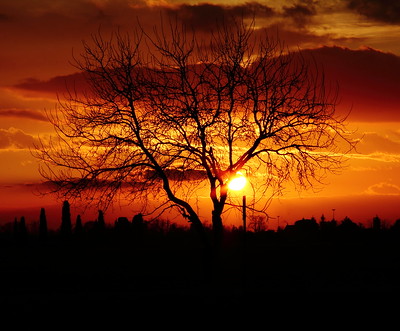A striking sunset illuminates this image, featuring a large, leafless tree with branches extending to the top and sides of the frame. The bright, orange sun is centered behind the tree, casting its light through the thin, wiry branches, which appear silhouetted and almost aflame with the sun's golden yellow, orange, and red hues. The sky is filled with clouds, darkening slightly at the top with hints of black, yet vibrant and brightened by the sunset’s glow. Below the tree, the ground is barely visible, shrouded in shadow with small rounded objects protruding, adding an eerie touch. A narrow black pipe stands out, nearly intersecting the sun's position. The entire scene, with its dramatic lighting and striking contrasts, resembles a piece of art, suitable for display in a home.